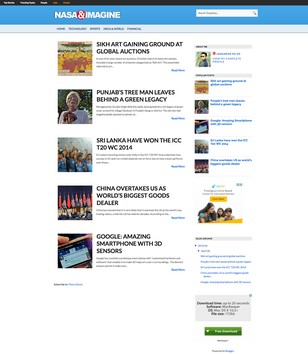A laptop screen displays a website, with the header featuring a horizontal blue bar at the top that includes a search dialog box and the words "NASA and Imagine." Below the header, the webpage showcases a series of news article headlines arranged vertically. Each headline is accompanied by a small square picture on the left. To the right of these headlines, there are smaller sub-menus that contain links to additional articles. The overall readability of the website is poor, making it difficult to discern the details within the content.